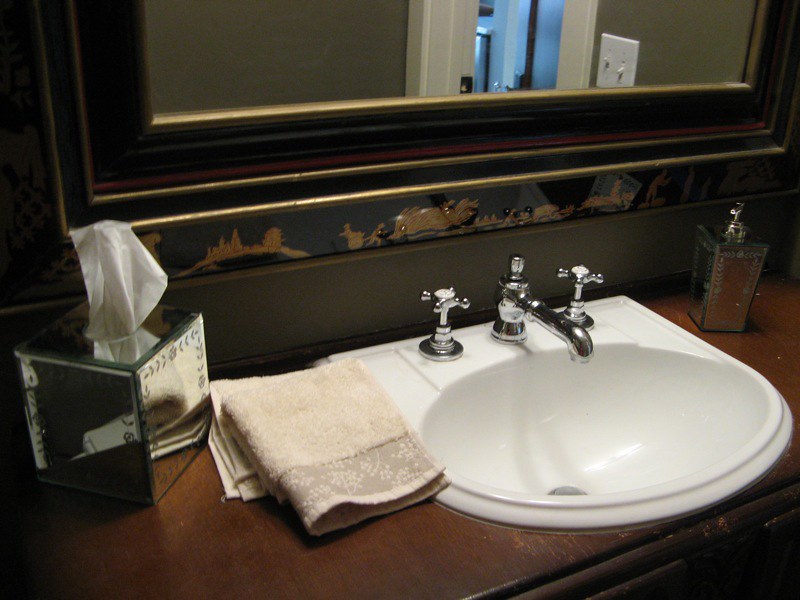A detailed view of an elegantly designed bathroom vanity. Central to the composition is a modern sink, complemented by an array of neatly arranged bottles and a sleek facial tissue dispenser. Two towels are casually draped beside the sink, adding to the lived-in feel of the space. Above the sink hangs a substantial mirror, its thick, multi-layered squared frame exuding understated elegance with a hint of complexity, measuring approximately six to eight inches in depth. The mirror reflects a glimpse of an adjoining hallway, including a door and a light switch. The lighting in the image is soft, emanating from an overhead source, casting a gentle glow that highlights the earthy green and brown tones dominating the bathroom’s decor. The overall ambiance is calm and inviting, though a touch more brightness could enhance the visibility of the room’s intricate details.